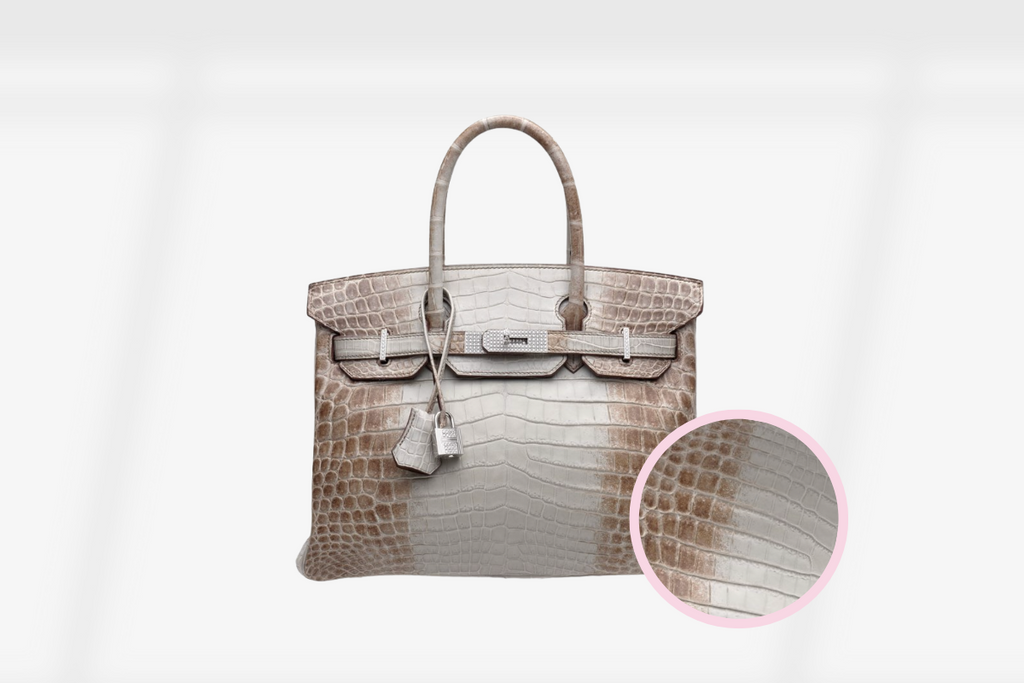This photo showcases a sophisticated purse against a clean white background. The purse, crafted from what appears to be animal skin—potentially snake or alligator—boasts a pearly iridescent white and light brown on some of the scales, exuding an elegant, luxurious feel. Its square shape is complemented by short, curved handles, rendering it quite practical as a clutch. A prominent feature is the silver buckle design that runs horizontally across the front, adding a touch of intrigue with three descending straps. An inset circular zoom-in highlights the intricate texture of the purse material, accentuating the detailed craftsmanship. Additionally, a petite lock and a matching tag dangle from the handle, contributing to its overall distinguished charm.